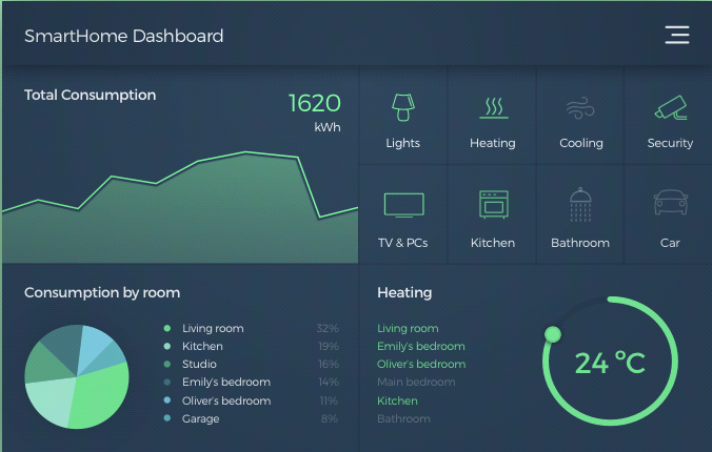The image depicts a detailed view of a smart home dashboard with a sleek black background. This central control screen allows users to manage various home functions such as lights, heating, cooling, security, TV and PCs, kitchen, bathroom, and car. Each function has its own interactive panel, where icons light up in green when active and remain shadowed when inactive. 

The top left section of the dashboard prominently displays the total energy consumption, measured in kilowatt-hours (kWh), with a line graph illustrating usage trends over time, showing fluctuations in energy consumption. Below this, a color-coded pie chart breaks down energy consumption by room, with sections indicating the living room at 32%, kitchen at 19%, studio at 16%, Emily's bedroom at 14%, Oliver’s bedroom at 11%, and garage at 8%.

On the top right, users can select specific areas of the home to monitor or adjust, including options for lights, heating, cooling, security cameras, televisions, computers, kitchen, bathroom, and car. The bottom left quadrant shows a graphical representation of energy usage by room, while the bottom right quadrant displays the current temperature in different rooms, all set to 24 degrees Celsius.

This smart home dashboard provides a comprehensive and user-friendly interface to efficiently monitor and control various aspects of home management, including detailed real-time data and visual aids for energy consumption and room temperatures.